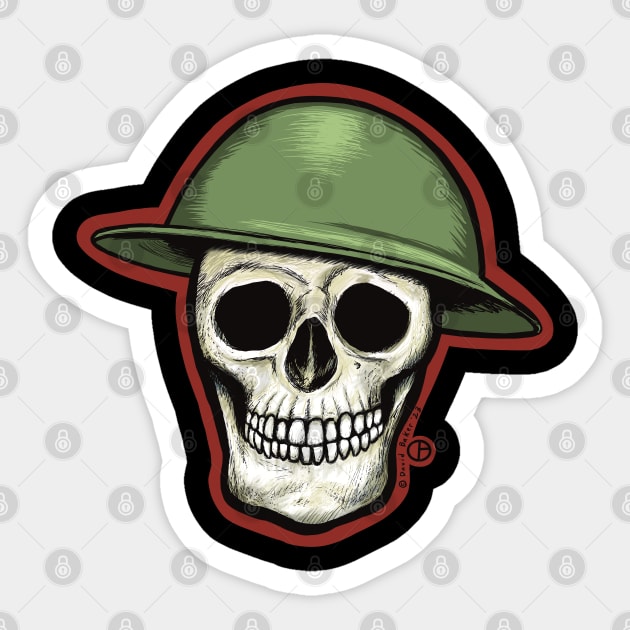The image depicts a white skull head with black eye sockets, a black nose, and a full set of exposed teeth, all outlined in layers of red, black, and white. The skull is adorned with a green, rounded army hat. The background of the image features a white canvas adorned with a pattern of circles connected by thin gray lines forming a diamond shape, with each circle containing a white lock symbol. The skull and hat are set within a central area outlined by a white border and a surrounding brown border, giving the overall image a digital or cartoonish appearance. Both captions emphasize the white skull head with black features and a green army hat, as well as the outlined layers and detailed background pattern.